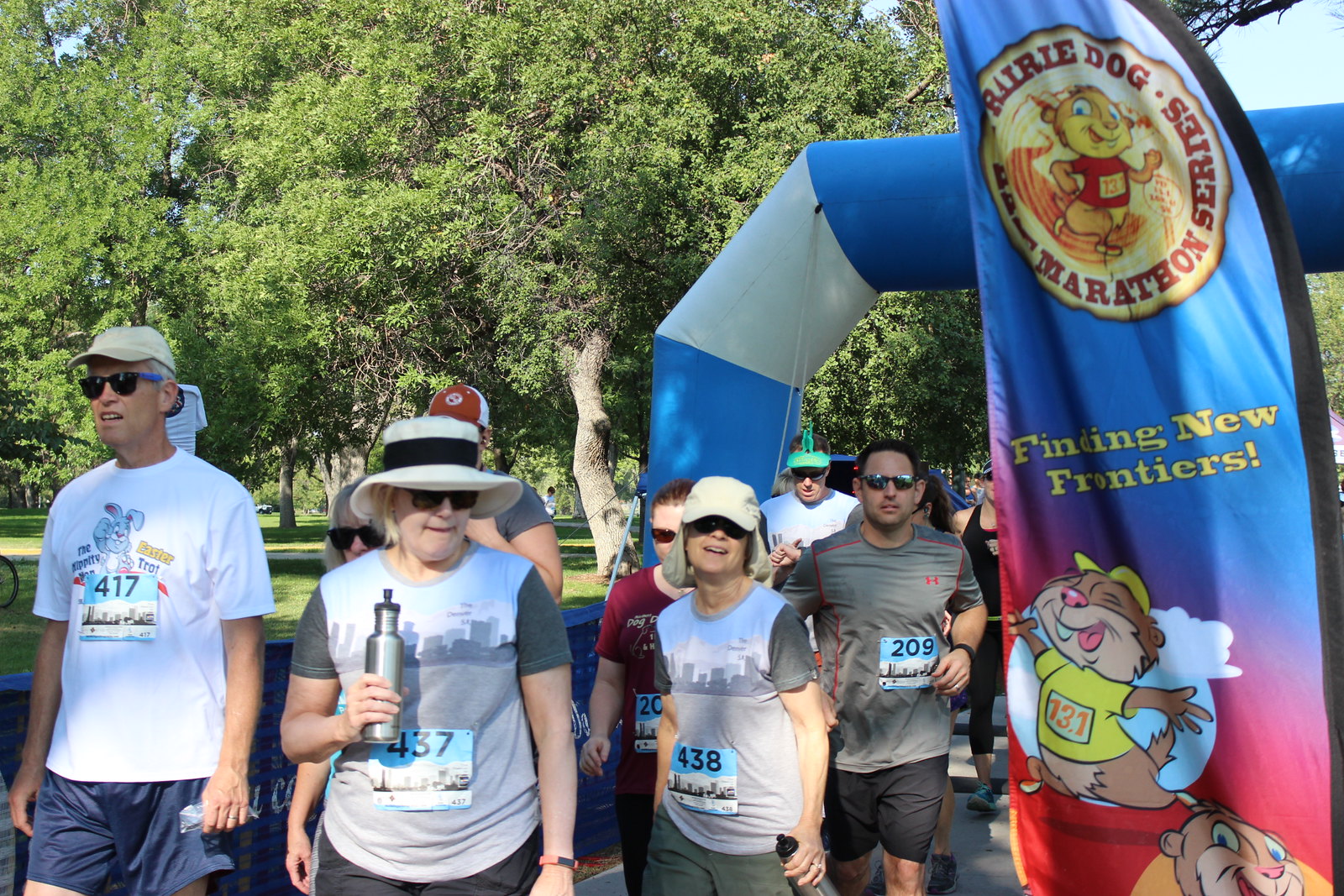In the image, a group of people appears to be gathered just in front of an inflatable blue and white barrier, marking what seems to be the finish line of a race. On the far left stands a middle-aged man in a white cap, black sunglasses, and a white shirt, with the race number 417 on a tag pinned to his shirt. To his immediate right is a woman wearing a straw hat with a black band and sunglasses. She dons a gray shirt featuring a city skyline print and holds a silver water bottle. Her race number, 437, is visible on a blue tag on her stomach. Standing next to her is another woman, wearing a cap pulled low over her eyes and sunglasses, with the same skyline shirt and a blue tag reading 438. To the right of her is a man with black hair, chromium sunglasses, and a gray shirt paired with dark black shorts. He also has a blue race tag displaying the number 209. The group is positioned near a flag on the right side, which has a logo at the top showing a cartoon prairie dog and the words "Prairie Dog Marathon Series." Below it, the tagline "Finding New Frontiers" is visible, along with a cartoon squirrel character dressed in a yellow hat and shirt, numbered 131. The scene is set on a bright day with clear blue skies, trees, and a lawn in the background. The smiling individuals, mostly wearing hats and sunglasses, seem excited and happy to be there, possibly after completing or in anticipation of participating in the marathon.